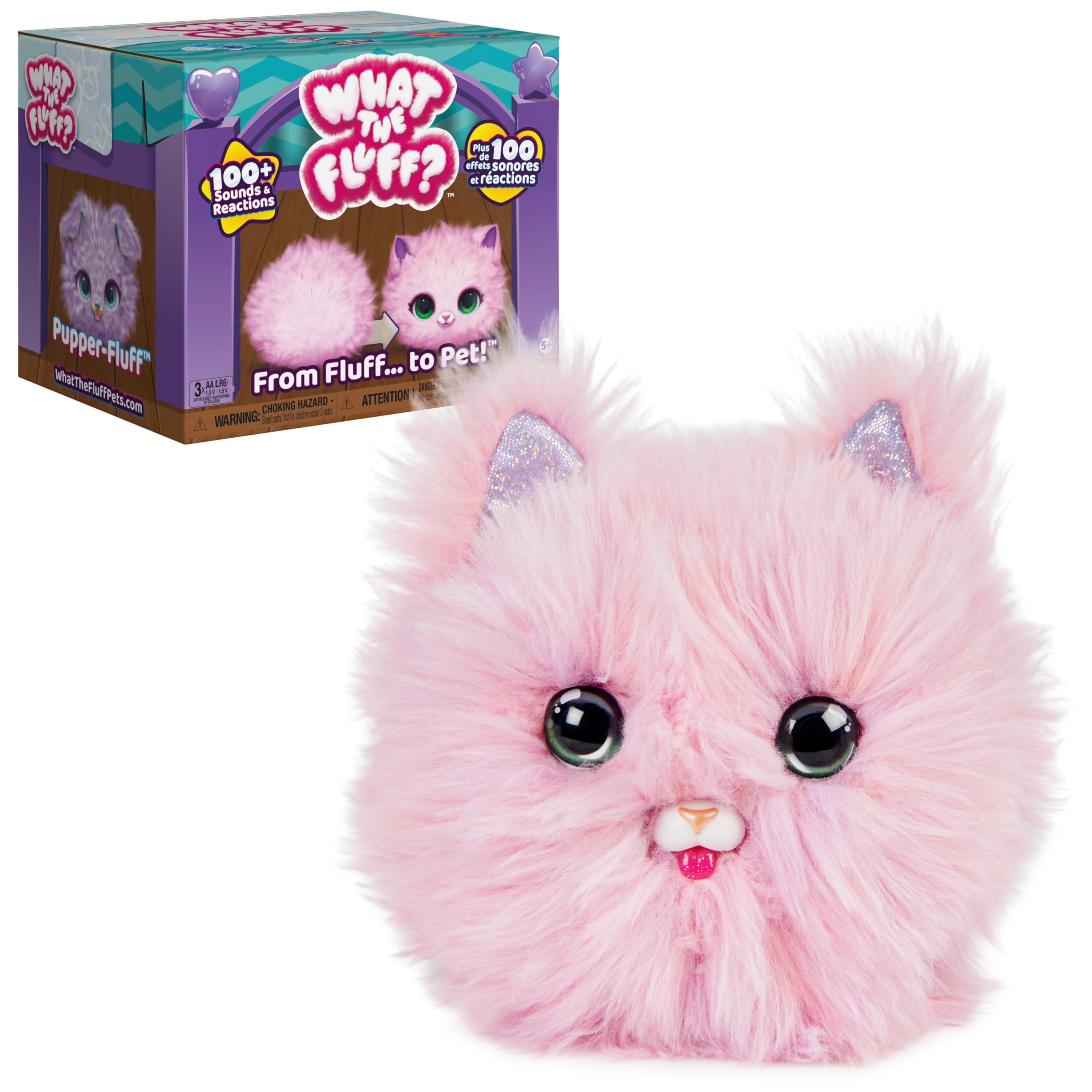This is an image of a children's toy that resembles a rounded, pink, fluffy cat. The toy's head, covered in soft fur, features large, round, marble-like green eyes that look directly at you. It has a tiny gold nose and a small mouth with a hot pink tongue sticking out. The toy also has two pointy ears adorned with purple accents and shiny sequined material. Behind the toy, to the left, there is a packaging box labeled "What the Fluff? 100 Sounds and Reactions. From Fluff to Pet." The box, colored in shades of purple and marine green, also showcases images of the toy and another character's head in purple, with text that reads, "Pup or Fluff?"